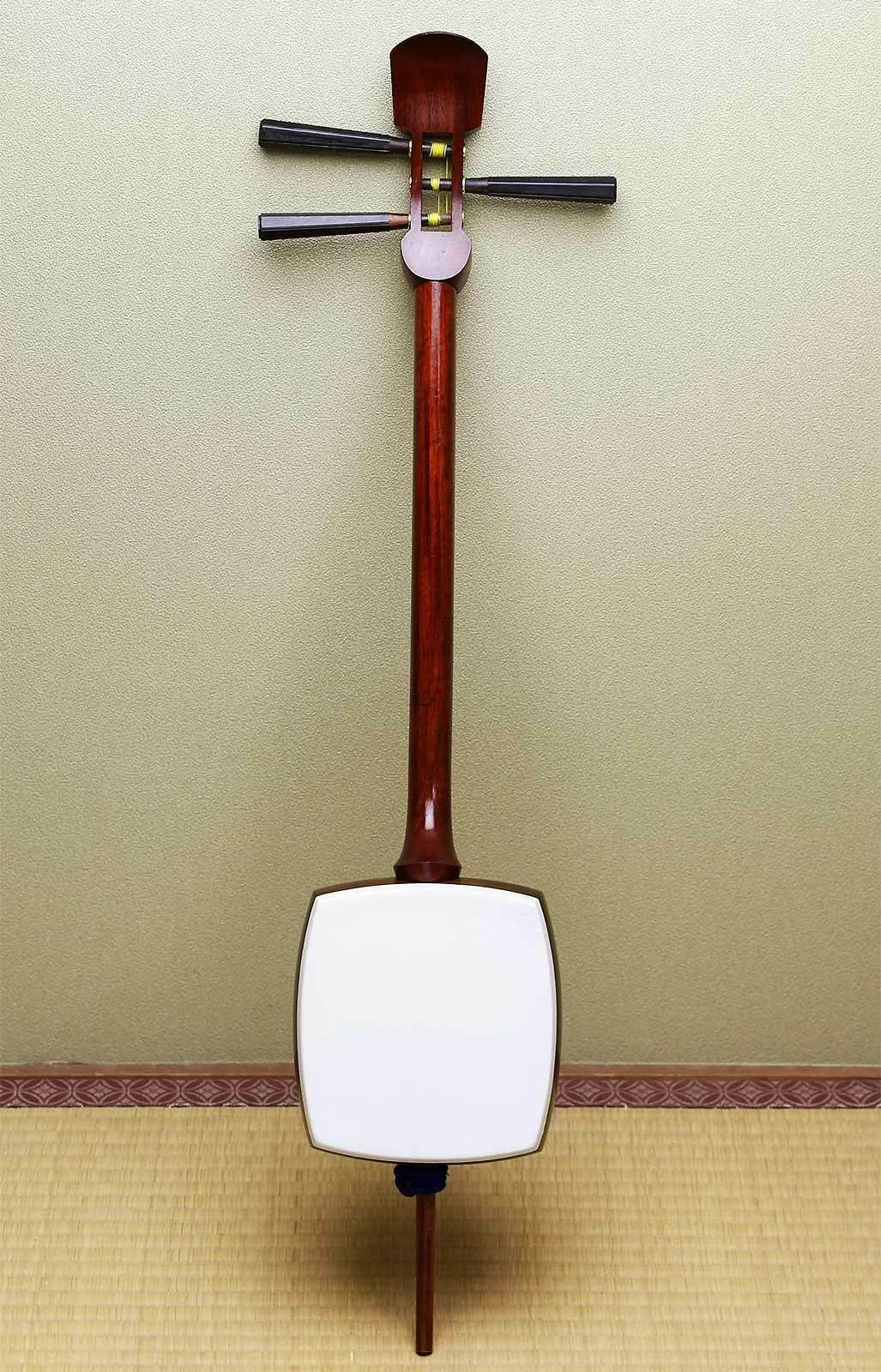The image depicts a peculiar object that closely resembles a musical instrument, such as a stringed instrument viewed from the rear. This object leans vertically against a light gray wall with a dark, ornamented maroon baseboard dividing the floor from the wall. The floor appears to be a light mocha brown with a square-ish pattern, similar to linoleum.

The instrument has a distinct design, featuring a long neck made of mahogany or reddish wood. At the top, there are three dark brown or black levers positioned two on the left and one on the right, possibly intended for tuning. These levers, augmented by what appears to be white strings wrapped around them, extend outward from a section resembling the head of a guitar, though no strings are visible, indicating it could be the back view.

The neck narrows down to meet a rectangular, slightly bloated white base at the bottom. This base is not perfectly square but has slightly curved edges, further sustained by a leg that contacts the ground. The overall composition of the image highlights the intricate and enigmatic design of the presumed musical instrument against its backdrop.